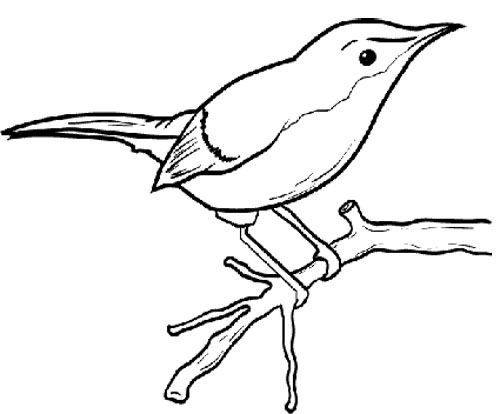This is a simple yet beautiful black-and-white line drawing illustration of a small bird, possibly a sparrow, perching on a branch. The background is entirely white, highlighting the stark contrast of the bird and branch outlines. The branch runs horizontally from the right side of the image, where it is cut off, towards the center but does not reach the left edge. The bird, with a rounded body and head, clings to this branch with its legs. It is oriented towards the upper-right corner of the image. You can see one prominent black eye, a thin curved beak, and long tail feathers extending straight back. This minimalist sketch captures the essence of the bird with its beady eye and distinctive shape, making it a charming, unembellished depiction.